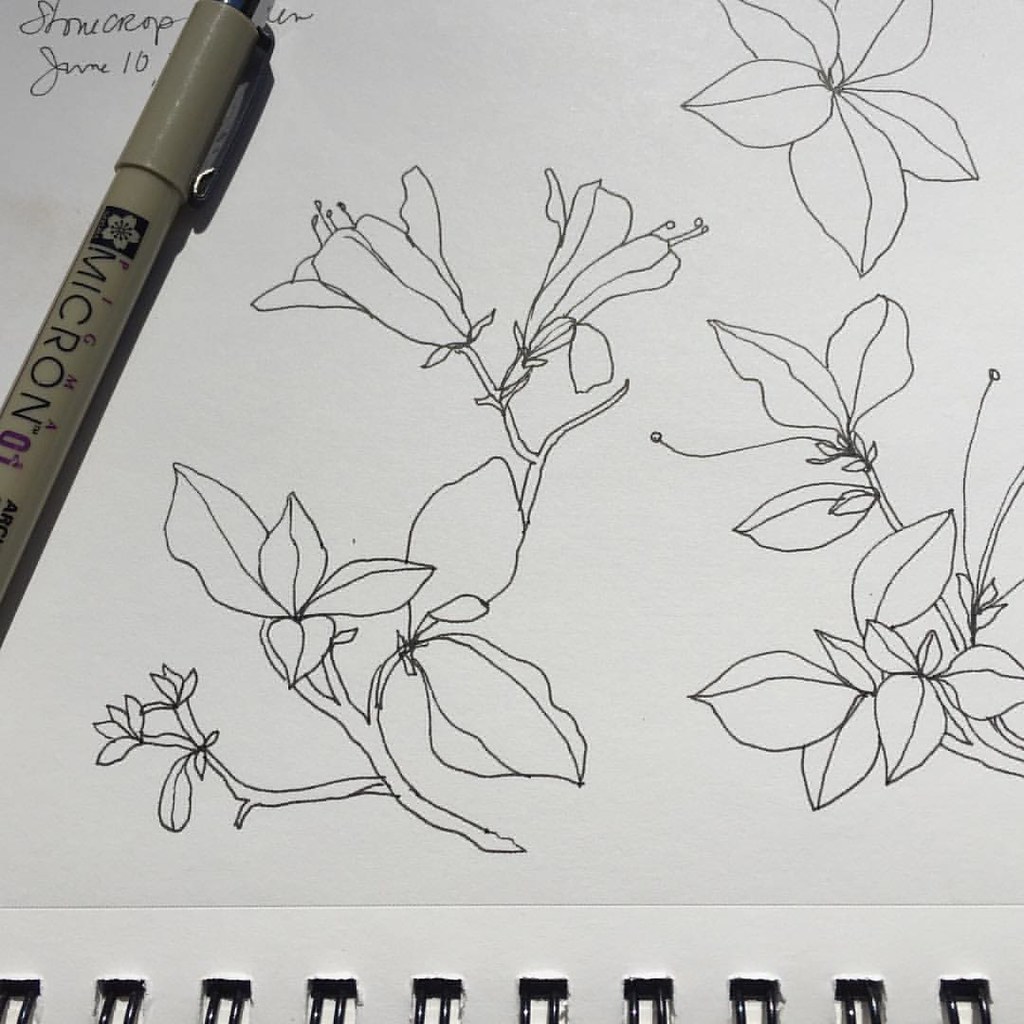A detailed, close-up photograph of a meticulously drawn botanical illustration, created with a fine-point black Micron marker, is displayed on a sheet from a white spiral-ring notebook, with the rings positioned at the bottom of the image. The marker itself, with a dark tan casing, is visible in the composition, although only part of its label, "M-I-C-R-O-N," is legible. 

On the upper left of the page, the title "Stonecrop" is elegantly inscribed in cursive, with some additional text partially obscured. Beneath the title, the date "June 10th" is clearly marked. The drawing features several branches and flowers of the same plant species, sketched in black ink without any color.

One prominent branch on the lower left showcases two flowers: one extending to the right and the other growing upwards. Another branch to the left displays three sets of small leaves and possibly a flower bud. Above, another flower is depicted in full bloom with five distinct petals, each marked by a single line running down its center and a cluster of stamens protruding from the middle. A side view of two blossoms further to the left reveals the receptacles beneath them and detailed filaments with anthers at the tips. Off to the right, an additional section of the same plant adds to the intricate composition of this black-and-white botanical study.